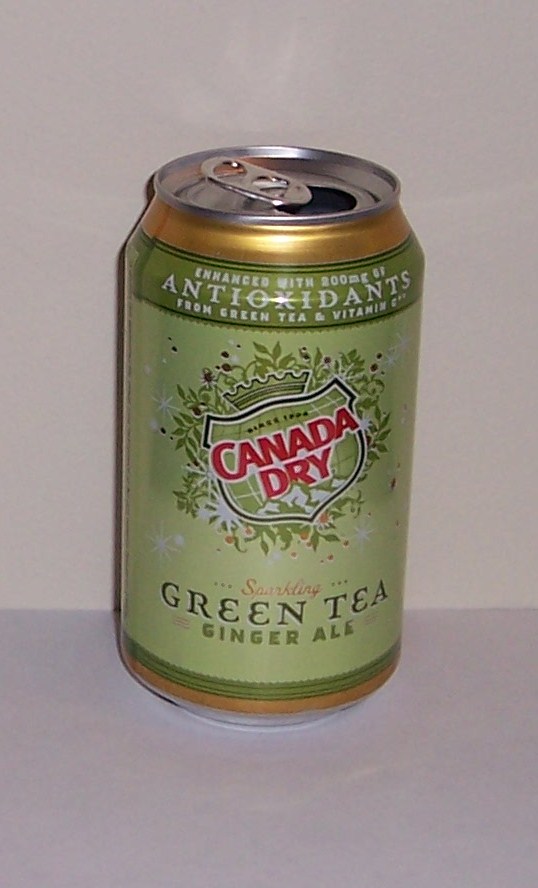This image features a Canada Dry Green Tea Ginger Ale can positioned on a dark gray countertop with a light tan wall in the background. The can's design includes a prominent light green center label with dark green font and a darker green border near the top. Both the top and bottom edges of the can are bordered in gold. The top of the can is silver with an open pop top. The front label displays the text "Canada Dry" in red letters, topped by the brand's crown logo. "Green Tea" is written in black letters, and "Ginger Ale" in green. The design incorporates small green leaves scattered across the light green background. A dark green banner just below the gold top border reads, "Enhanced with 200 milligrams of antioxidants from green tea and vitamin C."